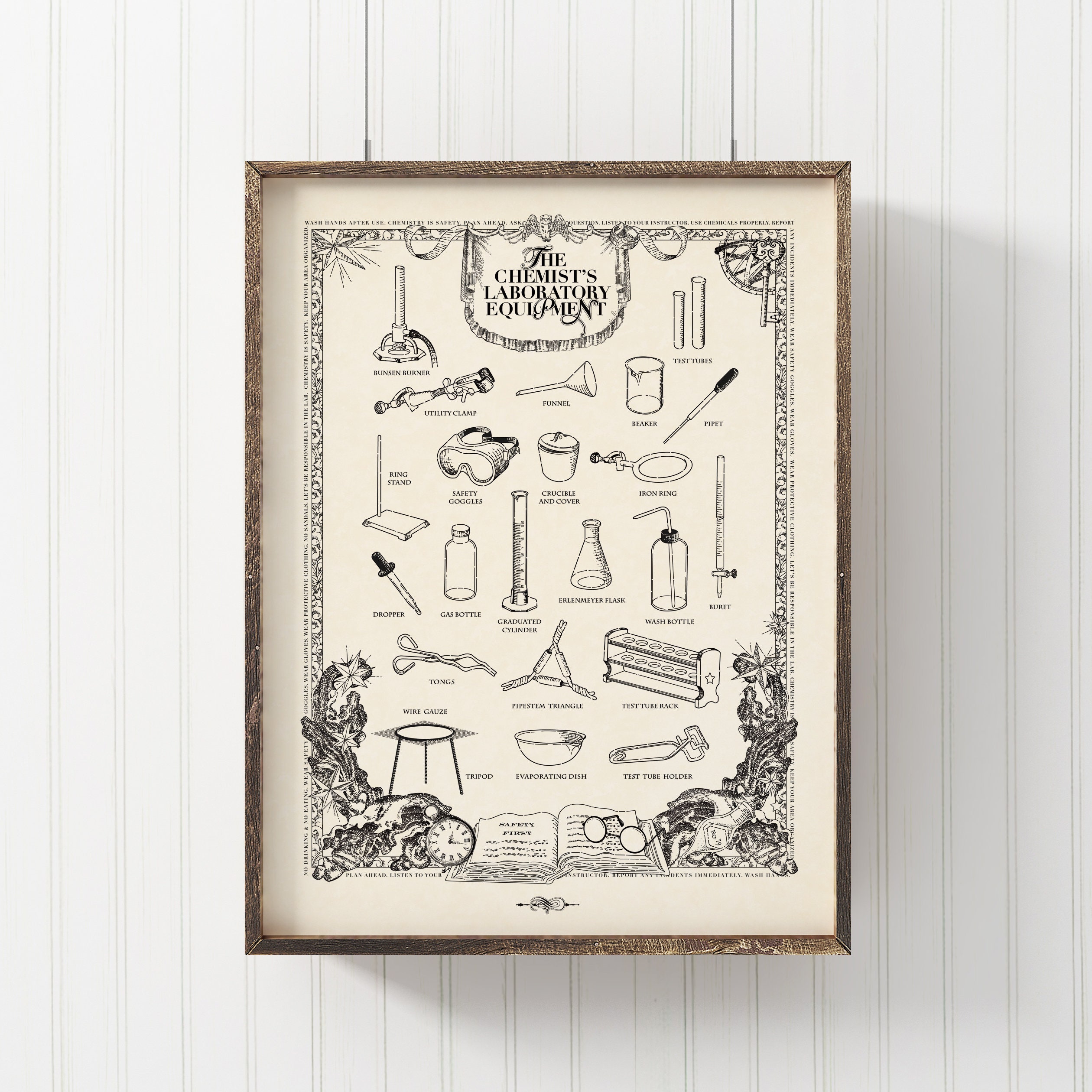The image depicts a framed sign hanging on a vertically paneled, beadboard-style white wall. The frame has a rustic, thin appearance, with a mushroom brown color. Inside the frame, an off-white background contrasts with black illustrations and text. The sign reads "The Chemist's Laboratory Equipment" at the top, and showcases meticulously drawn black-and-white images of various laboratory tools such as test tubes, a Bunsen burner, a beaker, a funnel, a dropper, and a tripod. These illustrations resemble items cut out from an old newspaper or magazine. The sign is bordered by a decorative black design and is suspended from the wall by two visible wires.